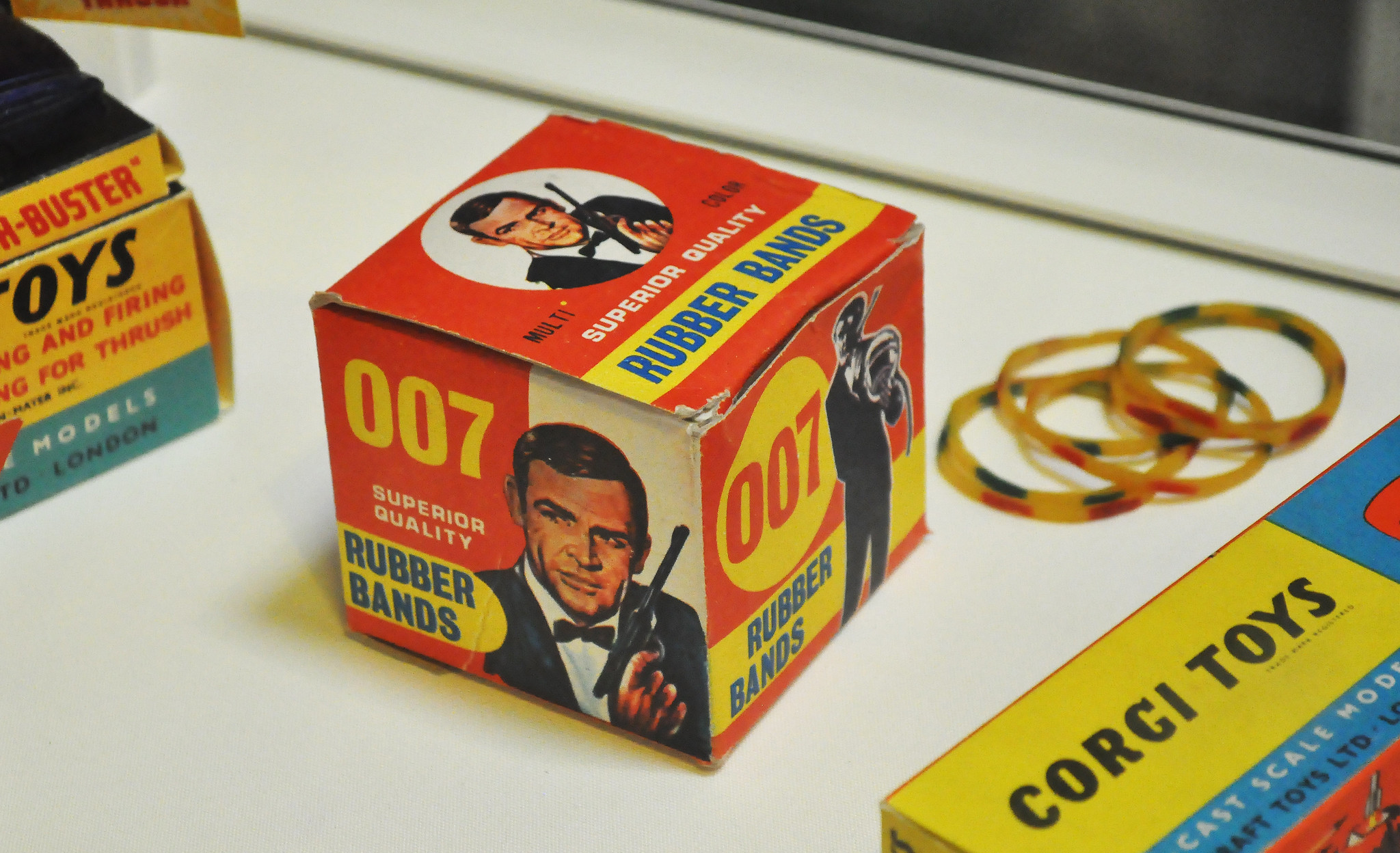This overhead landscape photograph captures a vintage-themed scene featuring several distinct objects on a white table. Central to the image is a small, old-fashioned cardboard box prominently displaying "007 Superior Quality Rubber Bands." The box is primarily red with a white circle on the top, showcasing an image of Sean Connery as James Bond, complete with a black suit, white dress shirt, black bow tie, and a pistol. The top of the box also features a yellow banner with blue print reading "Rubber Bands." The box's left side is divided into red and white sections with yellow print stating "007" and "Rubber Bands" again, along with another image of Connery's Bond. The right side is entirely red, featuring a yellow circle with "007" in red and a yellow band with blue lettering stating "Rubber Bands."

To the right of the 007 box, there's a small pile of yellow rubber bands with blue and red stripes. Adjacent to the rubber bands in the upper right corner, part of a yellow box with a blue bottom can be seen. This box has red print saying "Buster," black print saying "Toys," red print saying "Firing for Thrush," and "Models" in white on the blue portion with "To London" in black.

On the left side of the image, there’s a yellow box with a blue and red design labeled "Corgi Toys" in black. The scene suggests a collection of toys and items likely from the 1960s or 1970s, adding to the nostalgic atmosphere of the photograph.